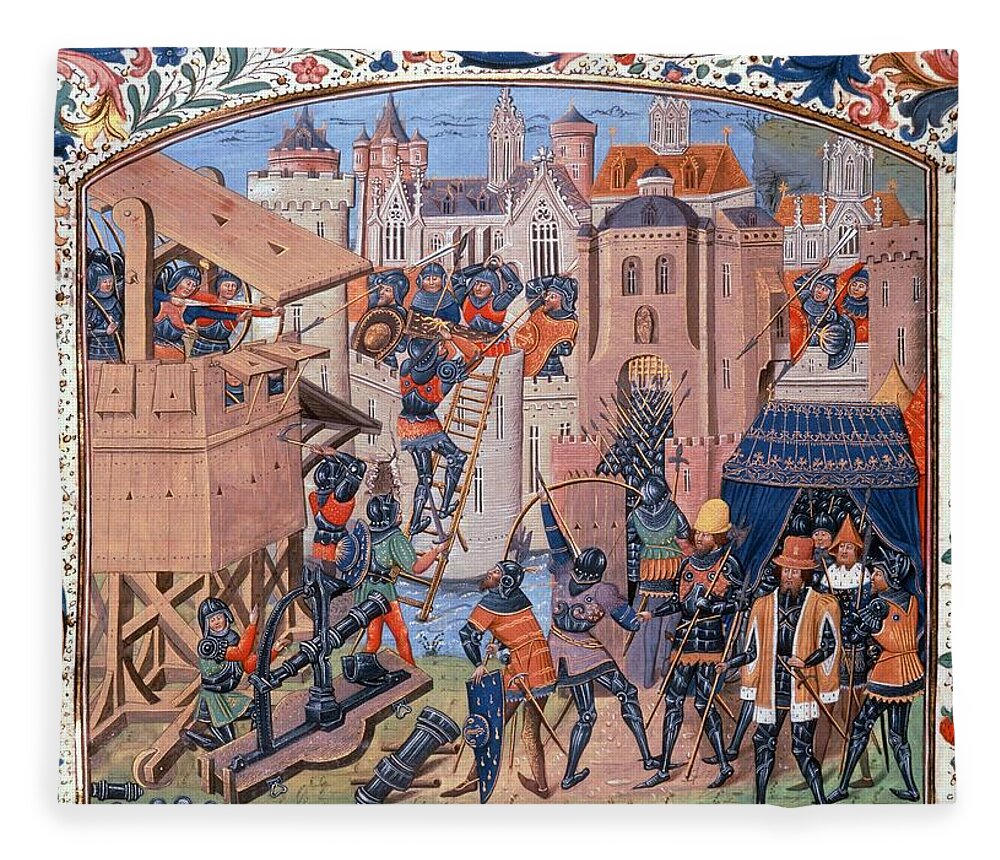The image is a detailed color painting with a landscape orientation, vividly illustrating a medieval battle scene, likely depicting the Hundred Years War between France and England. In the foreground, numerous soldiers clad in grayish-black metal armor and adorned with period uniforms and helmets are depicted. Some soldiers are seen wearing colorful robes—red and purple—over their armor, and a few oddly sport top hats with beards and brown hair. 

The soldiers, positioned mostly in the bottom right, are engaged with archers in a castle tower on the left side, and some are seen climbing a ladder propped against a beige castle structure to cross a body of blue water that resembles a moat. The soldiers on the ground are also managing a black metal cannon and some are using large, copper-colored shields to defend themselves. Meanwhile, archers atop wooden towers equipped with hinged overhangs are shooting arrows downwards. 

The cityscape in the background is dominated by Gothic-style castles and buildings with ornate towers and sharp peaks. The sky is a rich, winkle blue, adding to the vividness of the scene. Green land is visible in the distance to the right, adding depth to the painting.

Surrounding the image is an intricate border featuring red, yellow, and pink flower petals interwoven with green leaf vines, which adds a decorative, almost tapestry-like quality to the artwork. This combination of gothic architectural elements, detailed attire, and dynamic action offers a rich depiction of historical warfare in a vibrant, vintage historical art style.